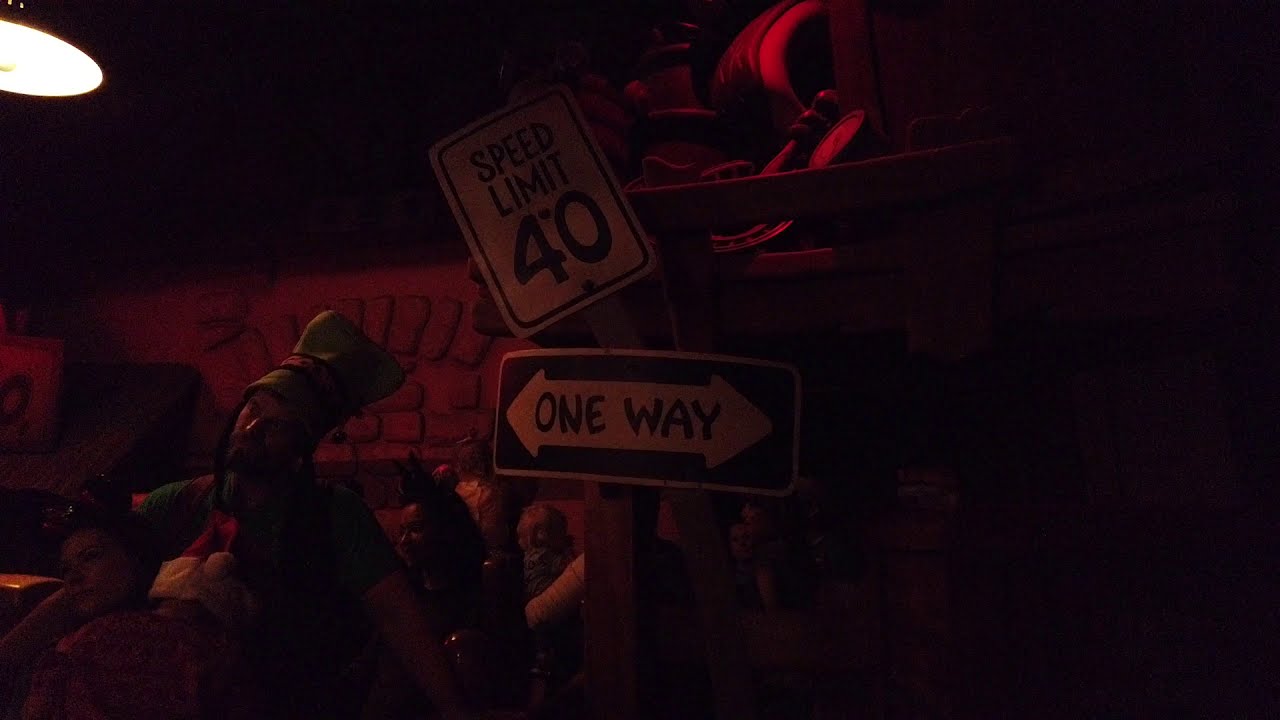In this dark, reddish-hued photograph taken inside a horror-themed amusement park attraction, we see a line of people, some in costumes, indicative of a themed event. The scene is partially illuminated by a lamp near the top right corner, casting a light on the eerie setting. Dominating the middle of the image is a wooden post adorned with two signs: a speed limit sign marked "40" and a peculiar one-way sign with arrows pointing both left and right. The setting includes a stone barrier along a walkway and various items scattered or mounted on a wall, further contributing to the cluttered, spooky ambiance. Notable details include a person in an elf costume and others dressed distinctly, though their features are challenging to discern in the dim light. The overall scene evokes a sinister, post-apocalyptic streetscape, complete with a nearby cement brick wall, suggesting a narrative of decay and haunting atmosphere.